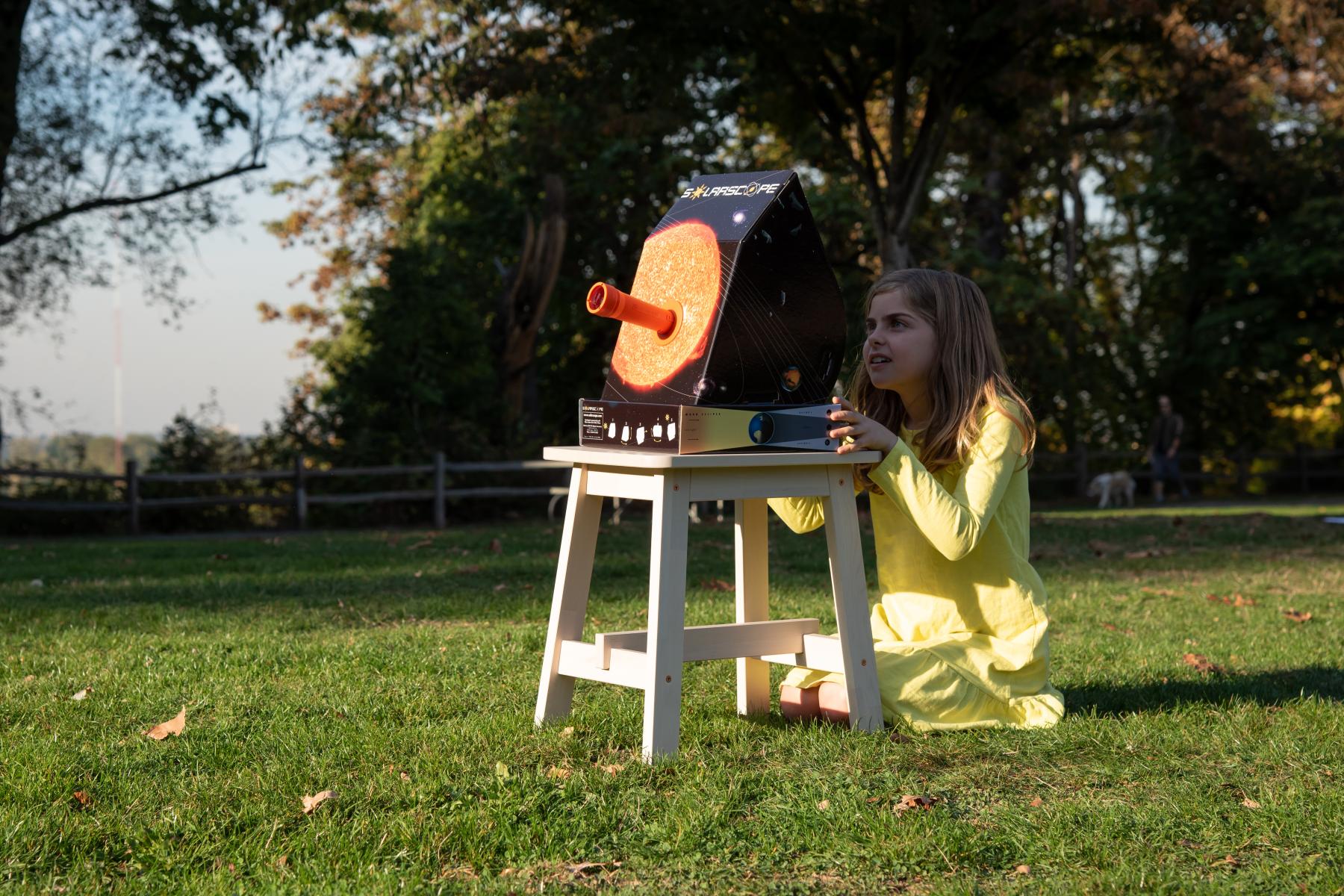In this color photograph taken outside during the daytime in a backyard, a little girl in a yellow dress sits on the grass near the front of the picturesque scene. She is engrossed in a homemade cardboard device designed for safely viewing the sun. This intriguing device, resembling a sun scope, is set on a small wooden stand and consists of a black cardboard box with a decorative image of the sun in orange on the front. An orange tube extends from the sun illustration, allowing a safe viewing experience, possibly indicating the box is intended for observing a solar eclipse. 

To the right, in the background, a man, who could be her father, is walking a large white dog along the log fence that stretches horizontally across the image. The yard is lined with trees, providing a partly shaded area in contrast to the sunny spot where the girl and her device are situated. The sky above is overcast, adding a soft light to the overall serene backyard scene. Additionally, the side of the black cardboard box features a colorful illustration of the solar system, showing planets in orbit, giving the scene an educational and whimsical touch.